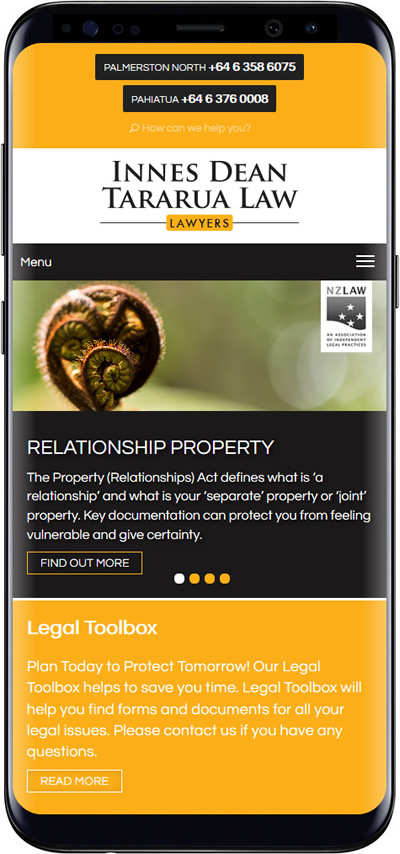The image prominently displays a modern smartphone with a sleek black design and curved edges. The left-hand side of the phone features both a long button and a smaller protruding button. At the top of the device, a faint line indicates the speaker, accompanied by what appears to be a small camera lens.

The screen of the phone shows a user interface with several elements. At the top, there's text displaying "Palmerstone North" followed by some numbers, and "Fiatu" with a similar numeric sequence nearby. Below this, an orange banner with a magnifying glass icon contains the prompt, "How can I help you?"

Underneath this orange banner lies a white section labeled "INSDEAN," followed by "Terura Law" and a headline in the middle stating "His Lawyers," also framed within small banners matching the top section. Further down, there's a menu section featuring an ambiguous image that resembles vegetation, alongside the text "NZ Law." Also visible is a topic labeled "Relationship Property" with an introductory paragraph and a prompt reading "Find out more."

Midway down the display are four buttons, one in white and the remaining ones highlighted in orange, labeled "Legal Toolbox." Below these buttons, another paragraph provides additional information with a prompt to "Read more."